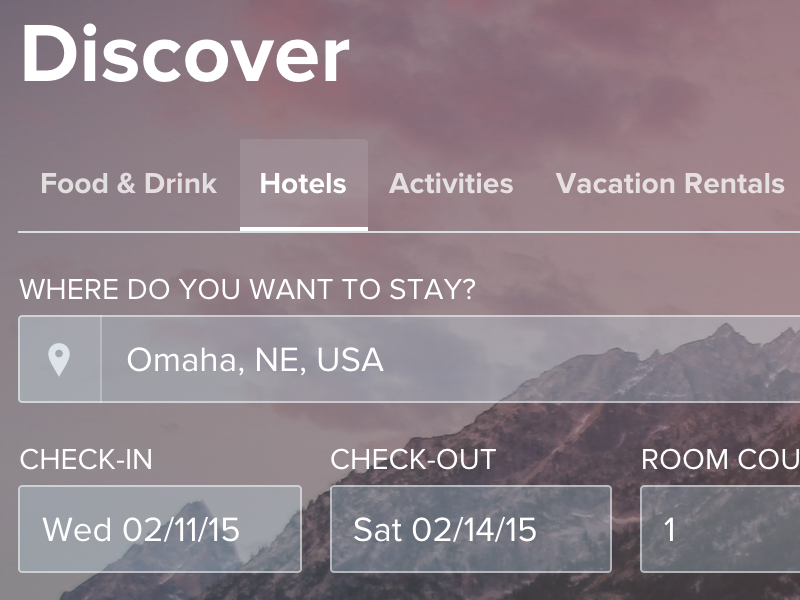The image is a slightly rectangular screen capture from a reservation website. At the top left, large white text reads "Discover." Below this header, a horizontal menu offers options including "Food and Drink," "Hotels," "Activities," and "Vacation Rentals." The "Hotels" option is highlighted with bold text and an underline. The next line asks, "Where do you want to stay?" followed by a field for inputting a location. Underneath, three fields are aligned side by side, labeled "Check In," "Check Out," and "Room Count." The lower left corner of the image features a pale, dusky pink background that extends diagonally upwards, fading into an intricate mountain range just below the center-right of the frame. The top portion of the image showcases a softly clouded sky, all bathed in the same pink hue, creating a serene and unified aesthetic.